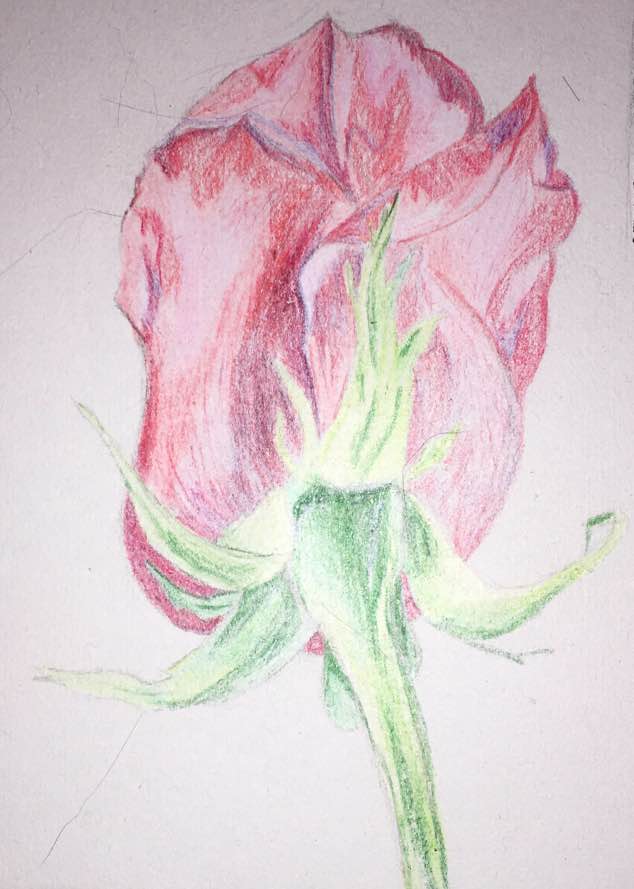This image showcases a beautifully detailed illustration of a red rose, which appears to be captured from a carefully rendered drawing done with colored pencils on a white sheet of paper. Dominating the composition is a large red rosebud that exhibits a stunning gradient of shades, ranging from deep, rich reds to softer pink hues, elegantly capturing the flower's natural beauty. The rosebud is perched atop a slender green stem adorned with several leaves, each skillfully shaded with varying tones of green, from dark forest hues to lighter, almost yellowish greens, adding depth and realism to the piece. The simplicity of the white paper background highlights the vivid colors and intricate details of the drawing, allowing the rose to command the viewer's attention. The meticulous use of shading and color variation throughout the rose and its leaves suggests a keen eye for detail and a high level of artistic skill.